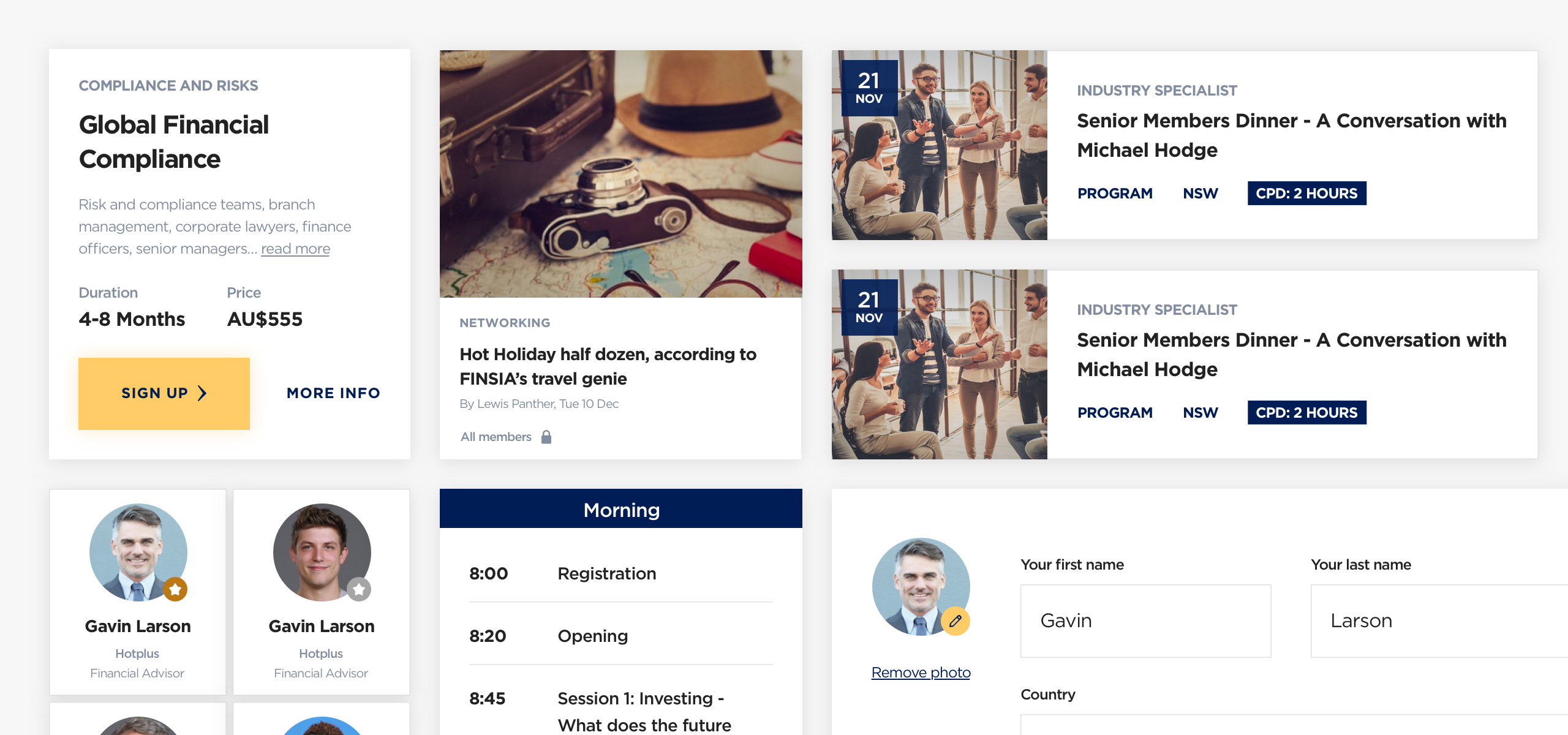This image is a detailed screenshot of a webpage belonging to a financial company. The website has a structured layout with a white background featuring various boxes and rectangles containing text and images.

In the upper left corner, the text reads: "Compliance and Risks: Global Financial Compliance." Below this heading, several roles are listed, including "Risk and Compliance Teams, Branch Management, Corporate Lawyers, Finance Officers, Senior Managers." Additional information indicates a duration of "4 to 8 months" and a price of "AU $555." A prominent yellow rectangle labeled "Sign Up" is clickable.

Beneath this section, there is a photograph of two financial advisors, both named Gavin Larson. The advisor on the left is an older white man with white hair and a smile, while the one on the right is a younger man with dark hair. The caption reads "Gavin Larson, Hot Plus Financial Advisor," suggesting that they might be father and son.

To the right of these images, a square displays a picture of an old camera, a hat, and a suitcase with the caption, "Networking: Hot Holiday Half Dozen According to Fincia's Travel Genie."

Below, a schedule outlines morning events starting with registration at 8 AM, followed by an opening session at 8:20 and a first session on investing at 8:45.

On the far right, there is an image of a group of people engaged in conversation. The accompanying text reads: "Industry Specialist: Senior Member's Dinner, A Conversation with Michael Hodge."

The overall impression is that the webpage is advertising a registration for a financial convention or a class led by these financial advisors.